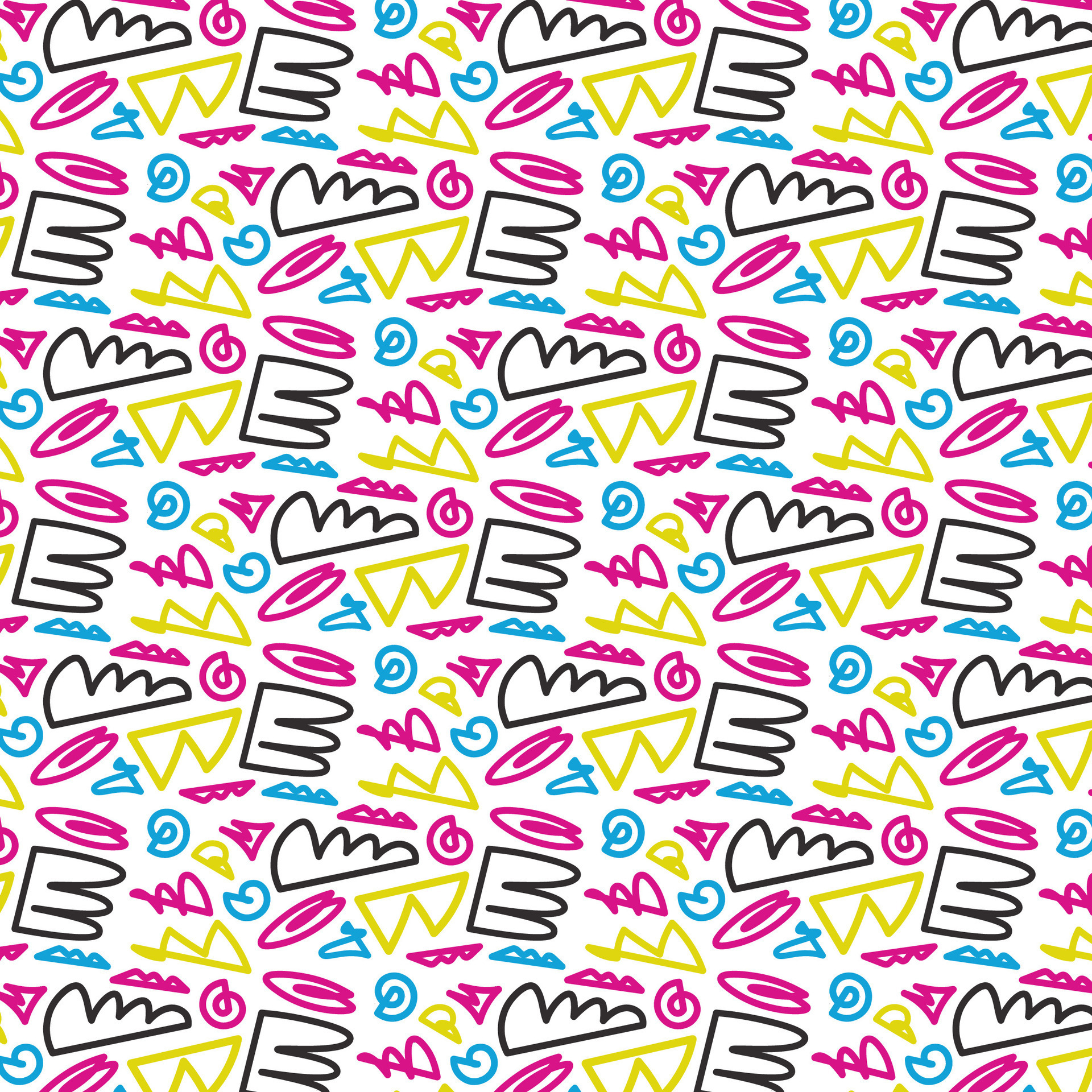The image is whimsical and consists of a repeating pattern of distinct, familiar shapes uniformly distributed across a white background. These shapes include black capital letter "E"s, yellow triangles resembling Dorito chips, teal "@" signs, and pink swirls. All shapes are outlined in their respective colors, leaving their interiors white. The overall design is both orderly and playful, creating a visually engaging and colorful scene.